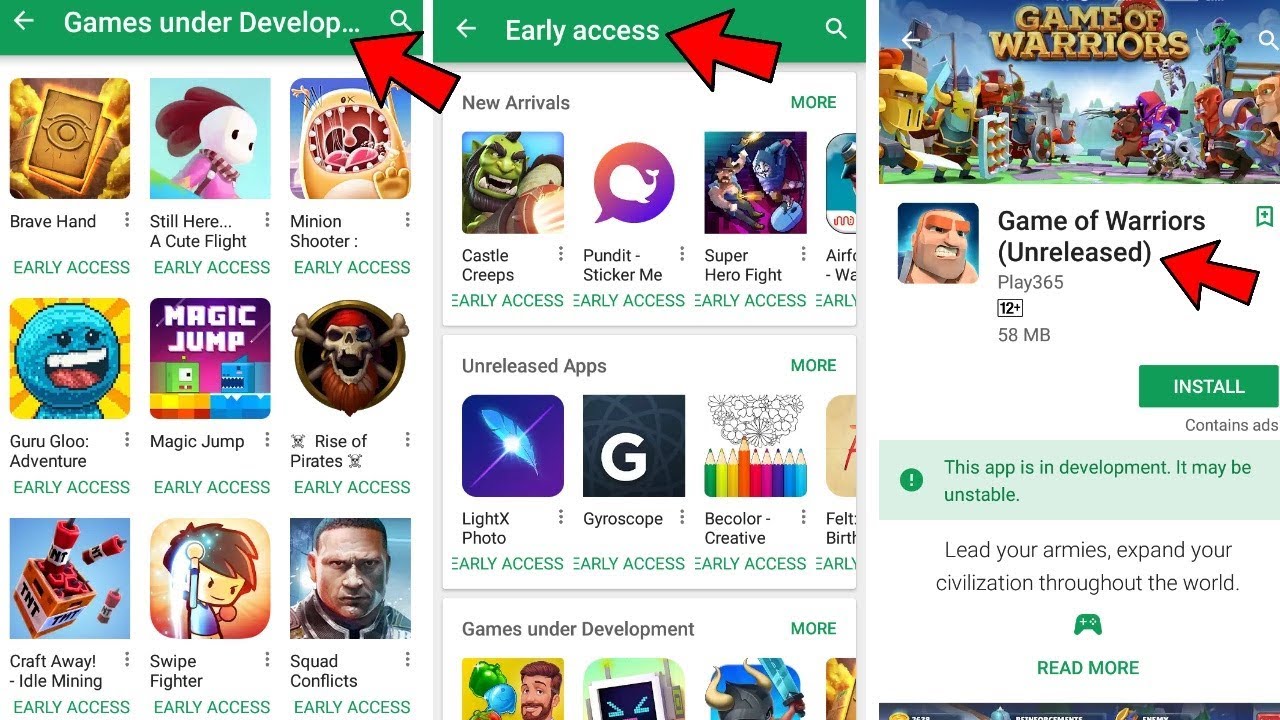The image showcases three consecutive cell phone screens displaying an app interface for a game under development. Each screen has a green banner at the top. 

On the first screen, the banner reads "Games Under Developed" with the text trailing off as "D-E-V-L-O-P..."
There is a backward arrow icon on the left and a magnifying glass icon on the right, both outlined in red with a black border. 

The second screen shows the same green banner but with the additional text "Early Access" at the top. 

The third screen highlights a game title "Games of Warriors" followed by the word "Unreleased" in parentheses, also in the same green banner. The red arrow points to this specific game.

Below the game title "Game of Warriors," detailed game information is listed:
- Publisher: Play 365
- Age rating: 12+
- File size: 58 MB

There is a prominent green "Install" button beneath the game details, accompanied by the note "Contains ads" in gray text. Below this is a light green band featuring a message: "This app is in development. It may be unstable." 

Further down, the text outlines the game's premise: "Lead your armies, expand your civilization throughout the world." An icon resembling either an open book or a game controller appears nearby, with the "Read More" link in green text. 

The color palette of the interface includes yellow, pink, brown, white, black, gray, blue, purple, red, orange, and various shades of green.